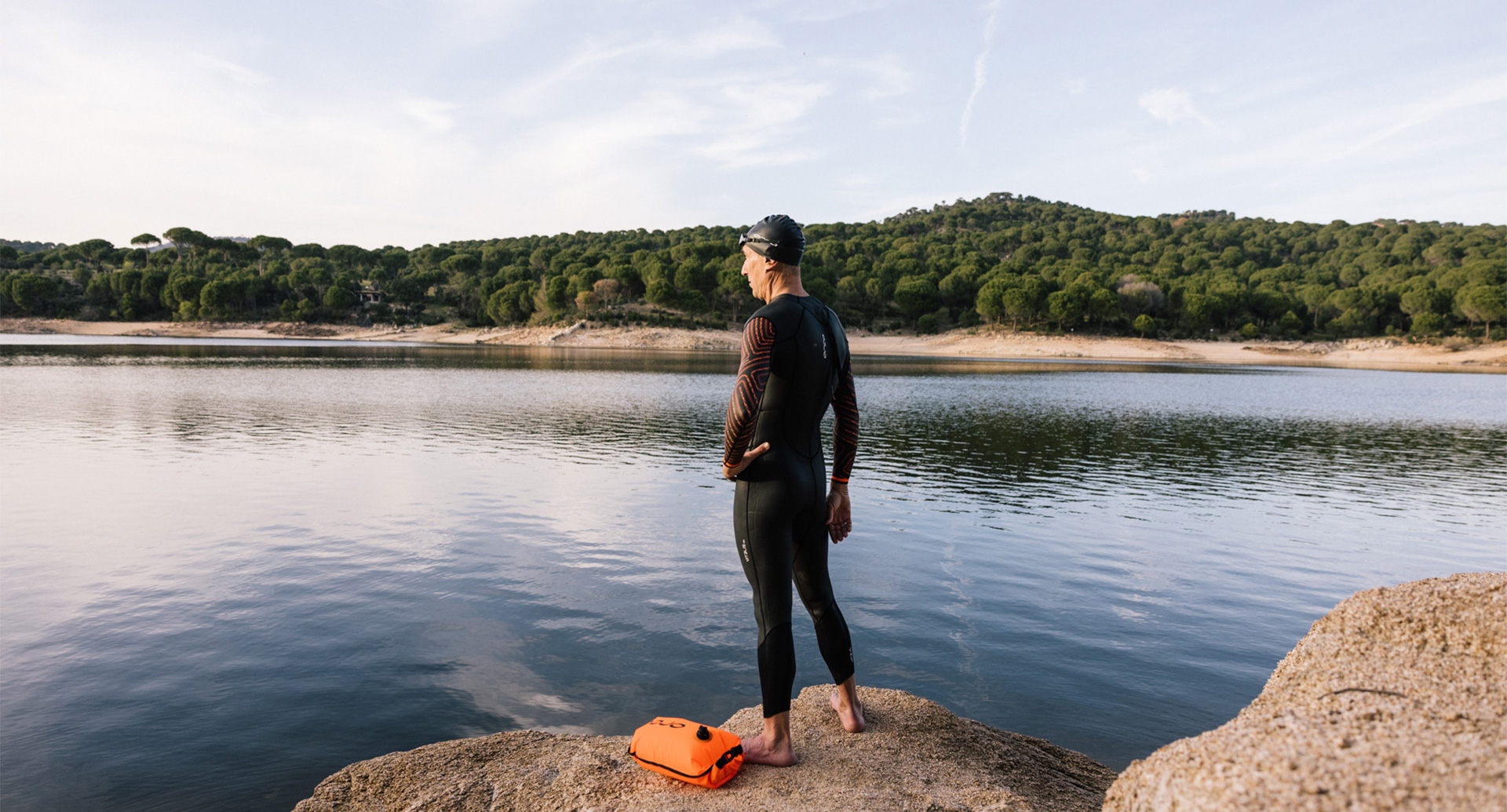In this image, a person is standing confidently on a large, beige boulder at the edge of a calm, dark blue lake. Dressed in a sleek black wetsuit with a glossy swim cap and goggles, they strike a poised stance with one hand on their hip and legs slightly apart, as if preparing to dive into the water. At the person's feet lies a small, orange inflatable pack, suggesting readiness for an aquatic adventure. The water below mirrors the sunlight, creating a striking gradient from dark blue to white. The backdrop features a dense tree line with rich dark green foliage, light brown sandy shores, and a hint of blue sky adorned with white clouds. An island with more trees and a mountainous area on the far left adds depth to the serene landscape.